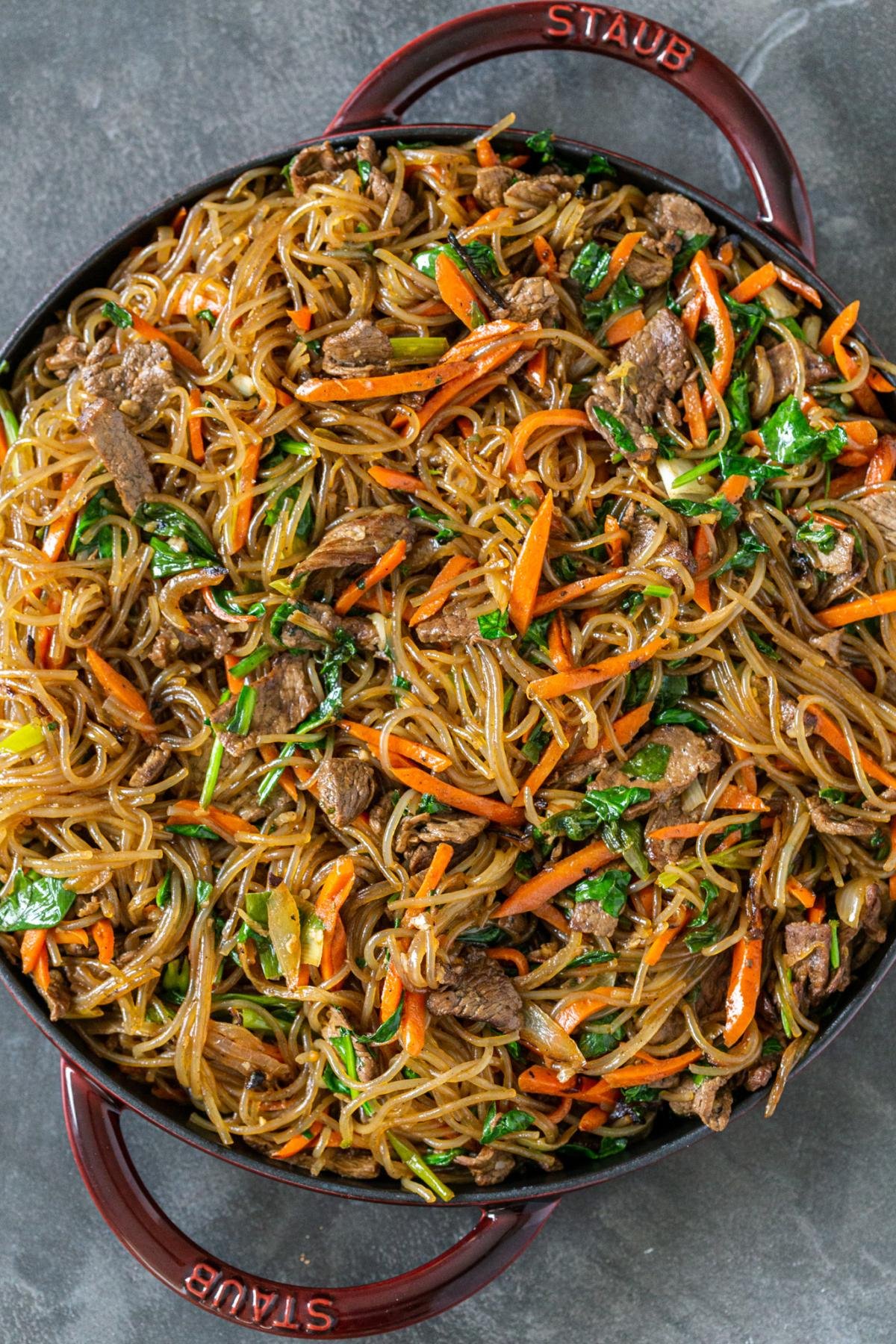The image showcases a vibrant and hearty stir-fry dish in a deep maroon red, round skillet with handles on both sides that are inscribed with the brand name "STAUB." The skillet, which appears slightly off-center in the image, is situated on a grayish-white granite countertop. The dish itself consists of clear stir-fried noodles, possibly Korean japchae or a variety of Chinese lo mein or chow mein, and is generously mixed with visible ingredients such as beef strips, carrot shavings, green leafy vegetables, and potentially some broccoli. The pan is brimming with this colorful, slightly oily, hearty mix, which extends close to the image's edges, giving a sense of fullness and abundance.